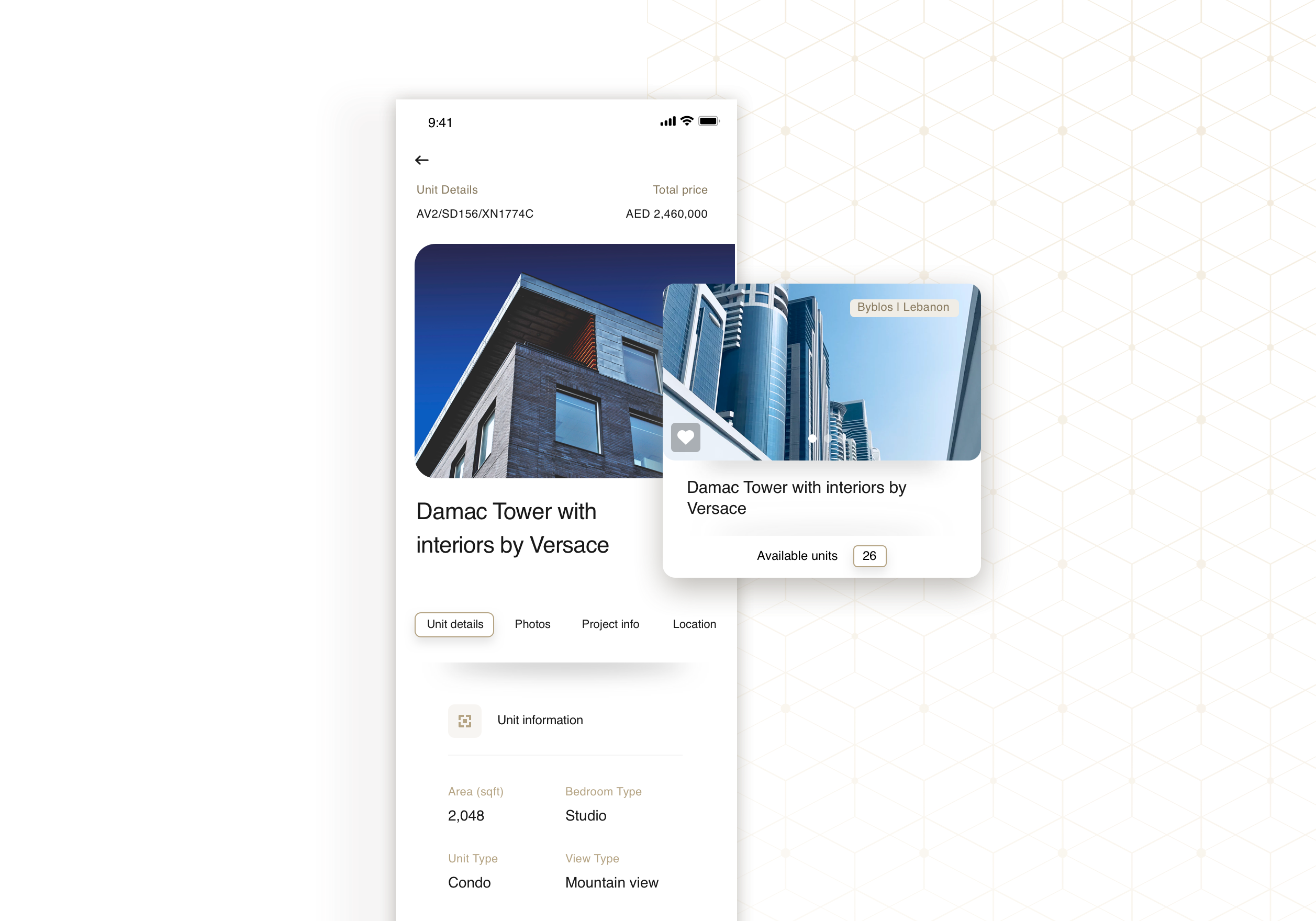The image is a collage-style screenshot taken from a smartphone, featuring content from two retail websites. The overall shape of the image is rectangular, with its width longer than its height. The primary screenshot is positioned towards the left side of the collage and occupies a larger portion of the space. Superimposed over this screenshot, slightly off-center towards the left, is a smaller screenshot from a similar website.

The main screenshot has a white background and includes the smartphone's user interface elements at the top. The top left corner shows the time '9:41', while the top right corner displays connectivity icons including a signal strength symbol, a Wi-Fi indicator, and a battery icon. Beneath the UI bar, brown text reads "Unit Details" and "Total Price," followed by black text which states: "AV at 2 / SD 156 / XN 1774C."

The background of the entire collage is white, adorned with multiple gold-bordered parallelogram shapes arranged to create a geometric pattern. This refined and structured background frames the screenshots and adds a modern, visually appealing aesthetic to the collage.